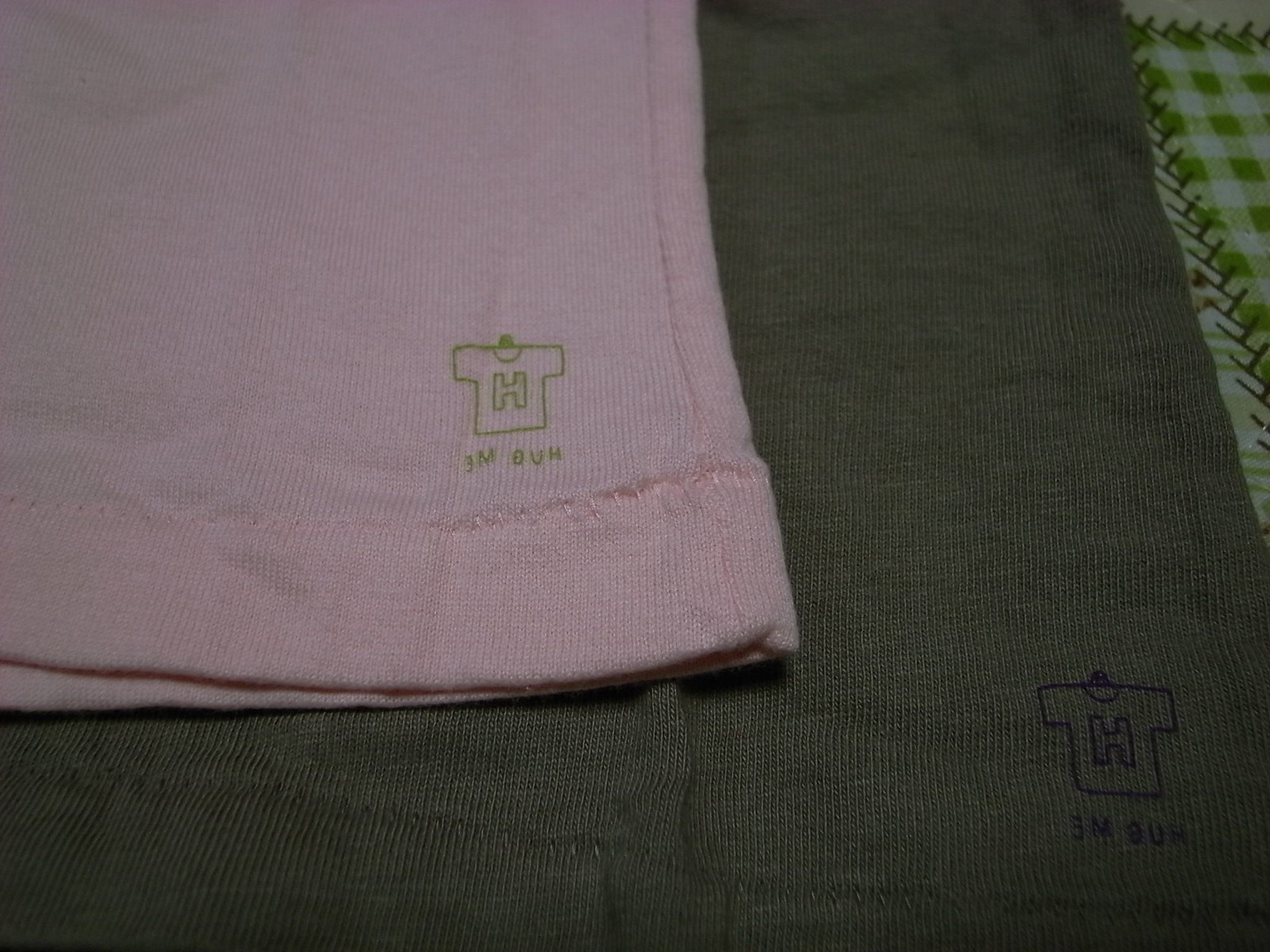The photograph depicts two articles of clothing arranged indoors on a quilted surface. The quilt features a white and green gingham check pattern, providing a charming and cozy backdrop. Laying neatly on this quilt are two t-shirts. The bottom garment, a gray t-shirt, only reveals its bottom corner. Positioned atop it, in a slightly angled manner, is a pink t-shirt, also showing its bottom corner. Both t-shirts exhibit a distinctive printed logo near their lower edges: an outline of a t-shirt encompassing the letter "H" in the center. Accompanying this logo are the letters "3MOUH," further adding to the specific branding detail. The overall composition and arrangement of the garments suggest a casual yet thoughtfully organized presentation.